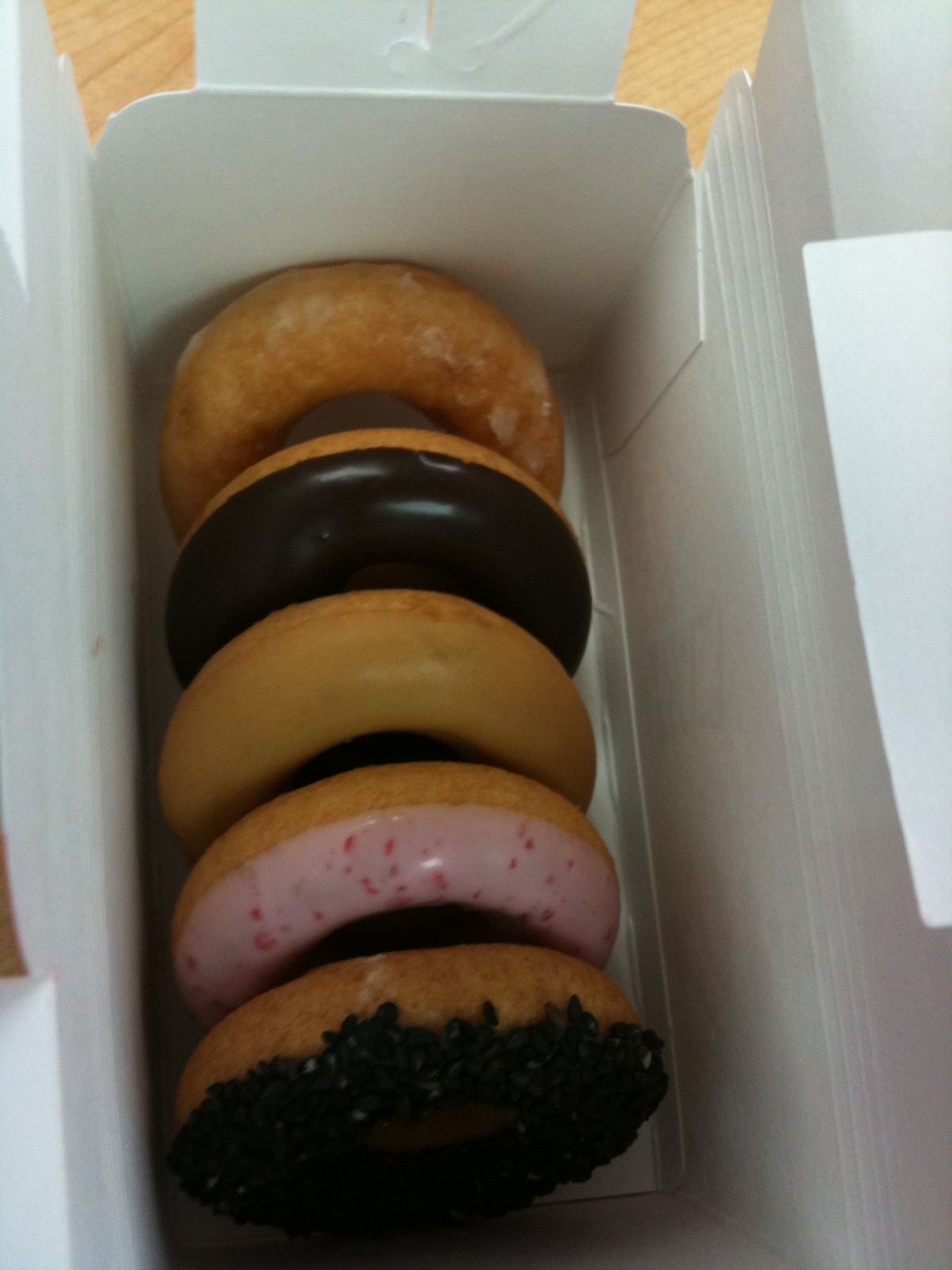In this detailed photograph, five donuts are intricately stacked on their sides within a unique white oblong takeout container. The container, which almost resembles an ice box due to its deep rectangular shape, is set vertically on a tan wooden table. The image provides a top-down view into the box, allowing us to appreciate the distinct textures and glazes of each donut. At the back, there is a cake donut with unusual glazing, hinting at its denser texture. Following it is a traditional donut with a rich chocolate glaze. In the middle sits a donut with a tan glaze that might be peanut butter. Next, a strawberry-glazed donut boasts a vivid pink color with red flecks, possibly tiny candies. At the front, a final donut is adorned with indulgent chocolate sprinkles over chocolate frosting, adding a layer of decadence to this sweet assortment.